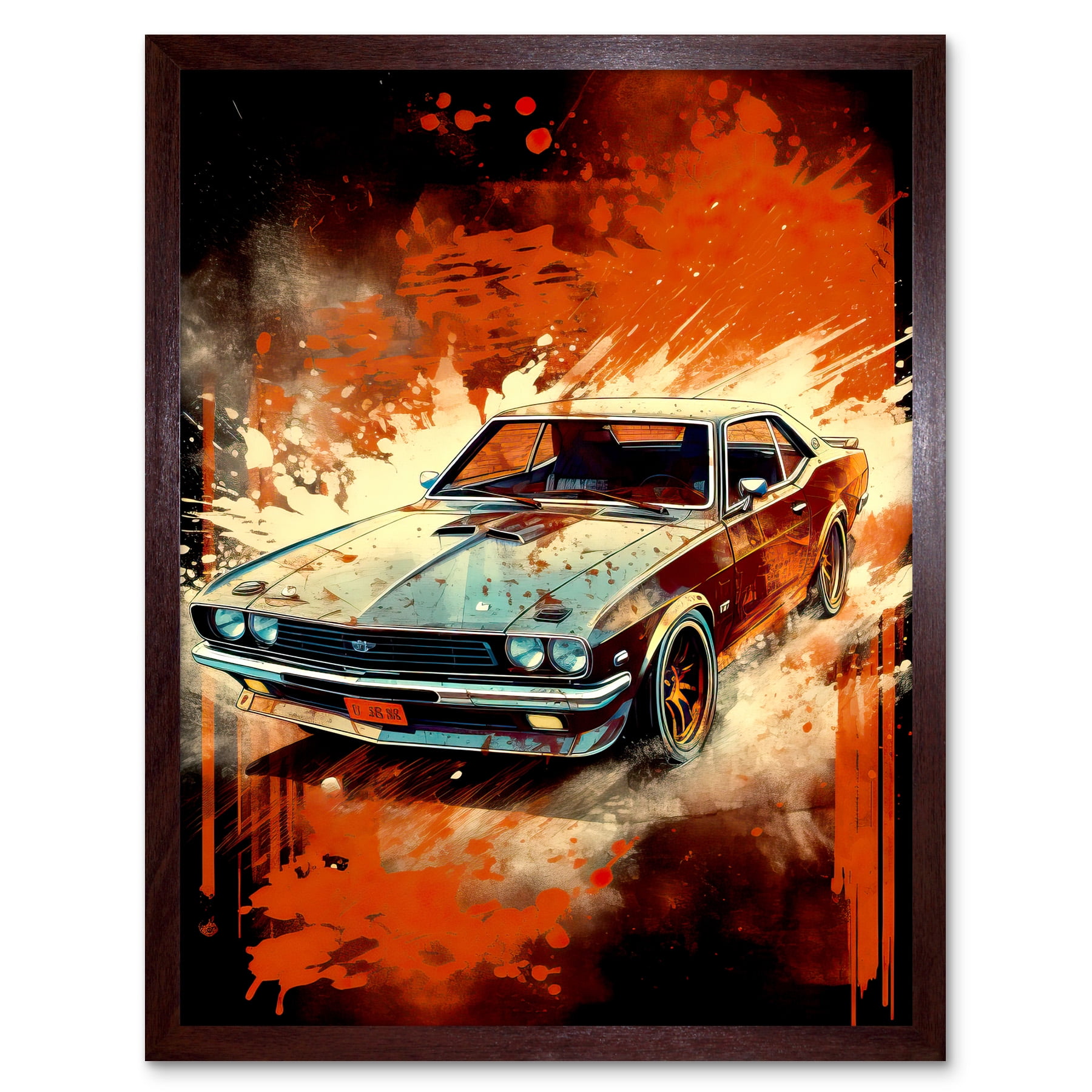The artwork depicts a vintage muscle car, likely a Camaro or a similar model, captured in a dynamic scene with splashes of vibrant colors. Set against a white wall and encased in a dark brown wooden frame that enhances the painting’s hues, the car is prominently displayed as a black two-door hardtop, showcasing its wide tires, silver rearview mirrors, and chrome bumper. The car's sleek body, potentially silver with red accents, contrasts with its black tires and orange-hued wheels. Visible details include red drips and splashes surrounding the vehicle, adding to the dramatic effect, with the car's red license plate serving as a focal point. Predominantly featuring colors such as black, dark brown, off-white, bluish tints, and intense reds, the painting exudes a vivid and striking portrayal of an iconic automotive classic.